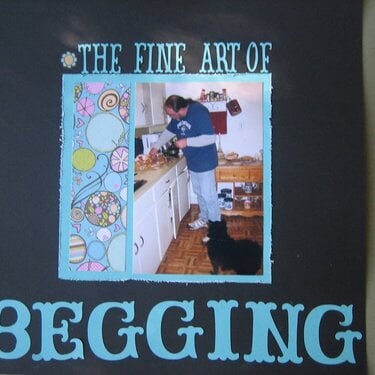The image titled "The Fine Art of Begging" features a man in his kitchen with a whimsical design and stylized text. The central photograph shows a man with long brown hair wearing a blue shirt over a gray long-sleeve shirt, blue jeans, and white sneakers. He is making a sandwich on a wooden countertop in front of white kitchen cabinets. A small black dog stands attentively next to him, clearly practicing the fine art of begging for food. The background has a black backdrop with the text "The Fine Art of" in smaller blue uppercase letters at the top left, featuring a dandelion design. The word "Begging" is prominently displayed at the bottom in large blue uppercase letters. To the left of the photograph is a whimsical, pastel-colored pattern featuring swirls, circles, and elements resembling dandelions or Easter decorations, enhancing the artistic and playful theme of the image.